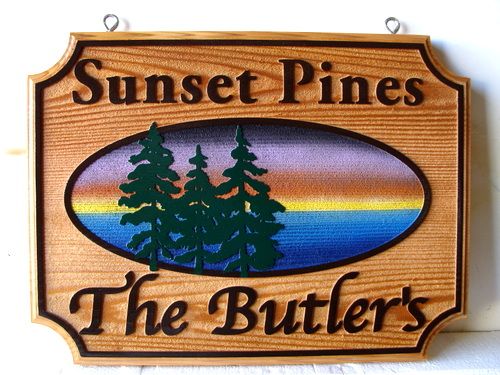The image depicts a detailed wooden sign, propped up against a white wall. The sign features two metal eyelet hooks at the top for hanging. At the top of the sign, the words "Sunset Pines" are carved in black serif font. Below this, there is an oval inset that contains an artistic depiction of three black pine trees. The background of the oval features a striking gradient, shifting from navy at the bottom, through cyan, yellow, and auburn in the middle, to lilac and violet at the top, mimicking a vibrant sunset. Beneath the oval, in a cursive script, are the words "The Butlers." The entire wooden plaque has an inverse beveled edge, framed by a black stroke perimeter. The scene is minimalistic, showing only the sign itself against a bit of white floor or table and a white wall, with a shadow cast by the sign adding depth to the composition.